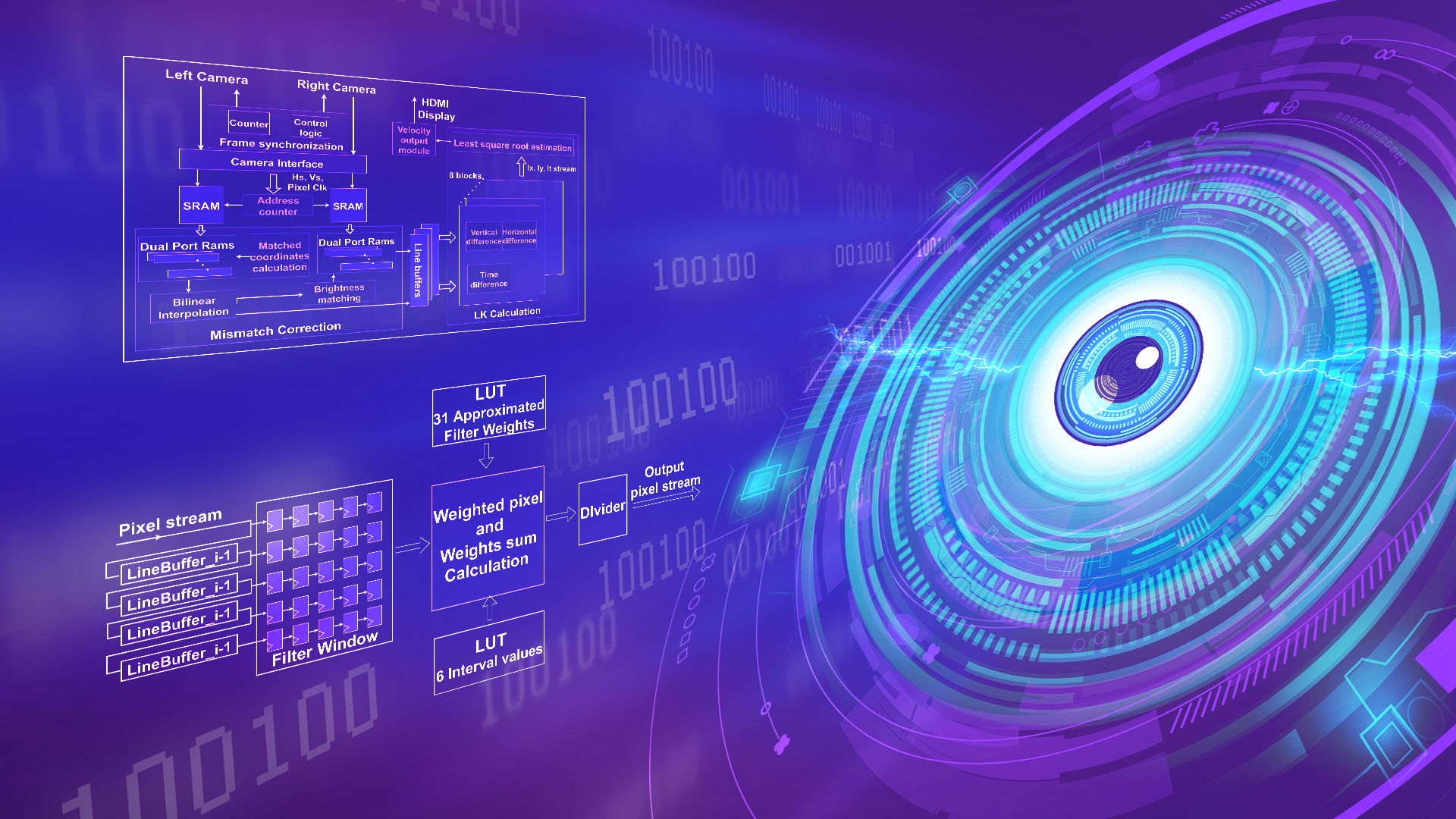This image is a computer-generated diagram that appears to illustrate a technological process, potentially related to video or photography. The background is predominantly purple with blue streaks running across it. On the left side, there is an intricate flowchart with multiple labeled boxes. The top box reads "Left camera, Right camera, HDMI display," followed by a series of connected boxes forming a comprehensive diagram. Among these boxes, there are headings like "Pixel Stream," "Filter Window" containing small square shapes, "LUT," "Weighted Pixel and Weight Sum Calculation," and "LUT Six Interval Values." Further to the right, the boxes indicate processes such as "Divider" and "Output Pixel Strength."

Dominating the right side of the image is a large, circular device resembling an eye. This 'eye' features a central dark purple/gray area with an inner white border, surrounded by progressively lighter blue circles and thin white borders. These circles extend outward until merging with a broad purple border that spans from the upper right corner to the lower middle of the image. The detailed flowchart on the left and the striking circular pattern on the right together create an elaborate and visually compelling depiction of a digital or technological concept.